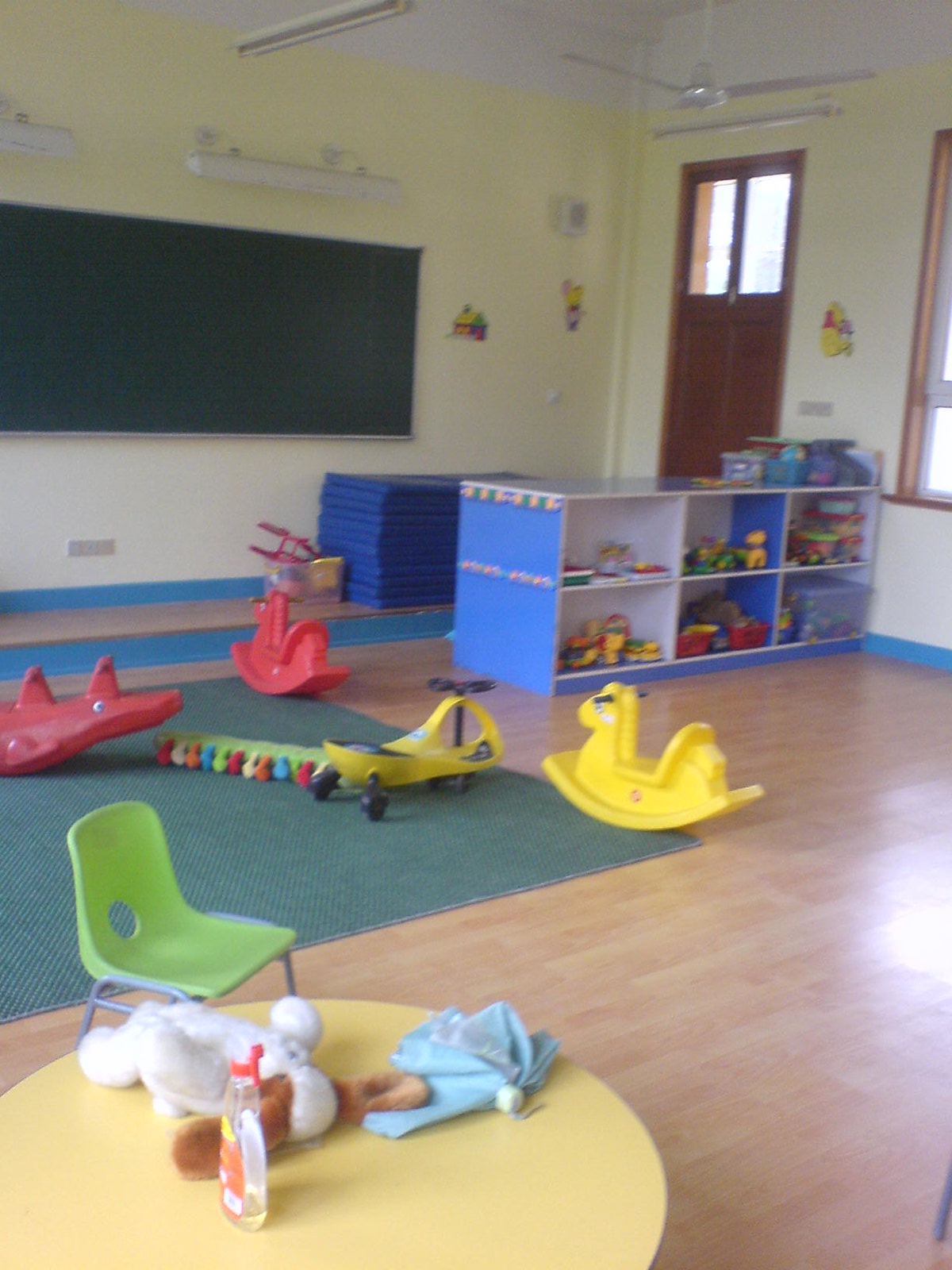This vertically aligned rectangular photo depicts a slightly blurry preschool classroom, especially on the right side and background. The classroom features a chalkboard in the upper left corner on a pale yellow wall adorned with various knickknacks. The ceiling is white with a ceiling fan hanging in the upper right area, adjacent to a brown wooden door with two rectangular windows cut out at the top. Near the door are white and blue cubbies and shelves filled with toys. Scattered around the room are rocking horse toys in red and yellow, a small green children’s chair, and a scooter with four wheels and a steering wheel. There is an alligator rocking toy as well. In the center of the room lies a large gray rug, surrounded by light brown tile. In the lower left-hand corner sits a round table with several stuffed animals, including a bunny lying on its back with ears flopped to the side and paws lifted. Adjacent to the table is a shelf with six compartments housing small toys, a clear plastic bottle, and a blue umbrella.